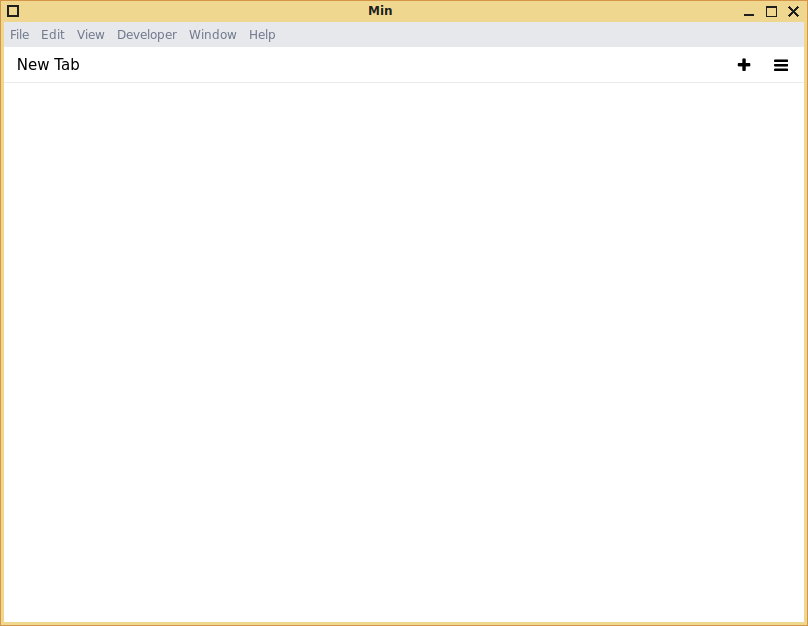The image depicts a pop-up window, prominently featuring a yellow color scheme with a yellow title bar and border. The title bar at the top contains three typical window control icons: minimize, maximize, and close. The title bar's header label reads "Min."

Beneath the title bar, there is a menu bar with several options including File, Edit, View, Developer, Window, and Help. The background of the screen under this menu bar is white with black text, which reads "New Tab" on the left side. On the far right of this menu bar, there is a plus icon and an icon of three horizontal lines, which usually indicate a menu with additional options.

The main content area of the window below the "New Tab" text is completely blank, featuring a white background. A horizontal gray line separates the menu bar from the main content area, likely serving as a visual divider which could replicate for additional rows if more items are listed. Despite the layout suggesting multiple features and functionalities, the window's primary function or the meaning of "Min" remains unclear based on the given details. The simplistic design and lack of content suggest it may be a template or an interface awaiting further input or configuration.